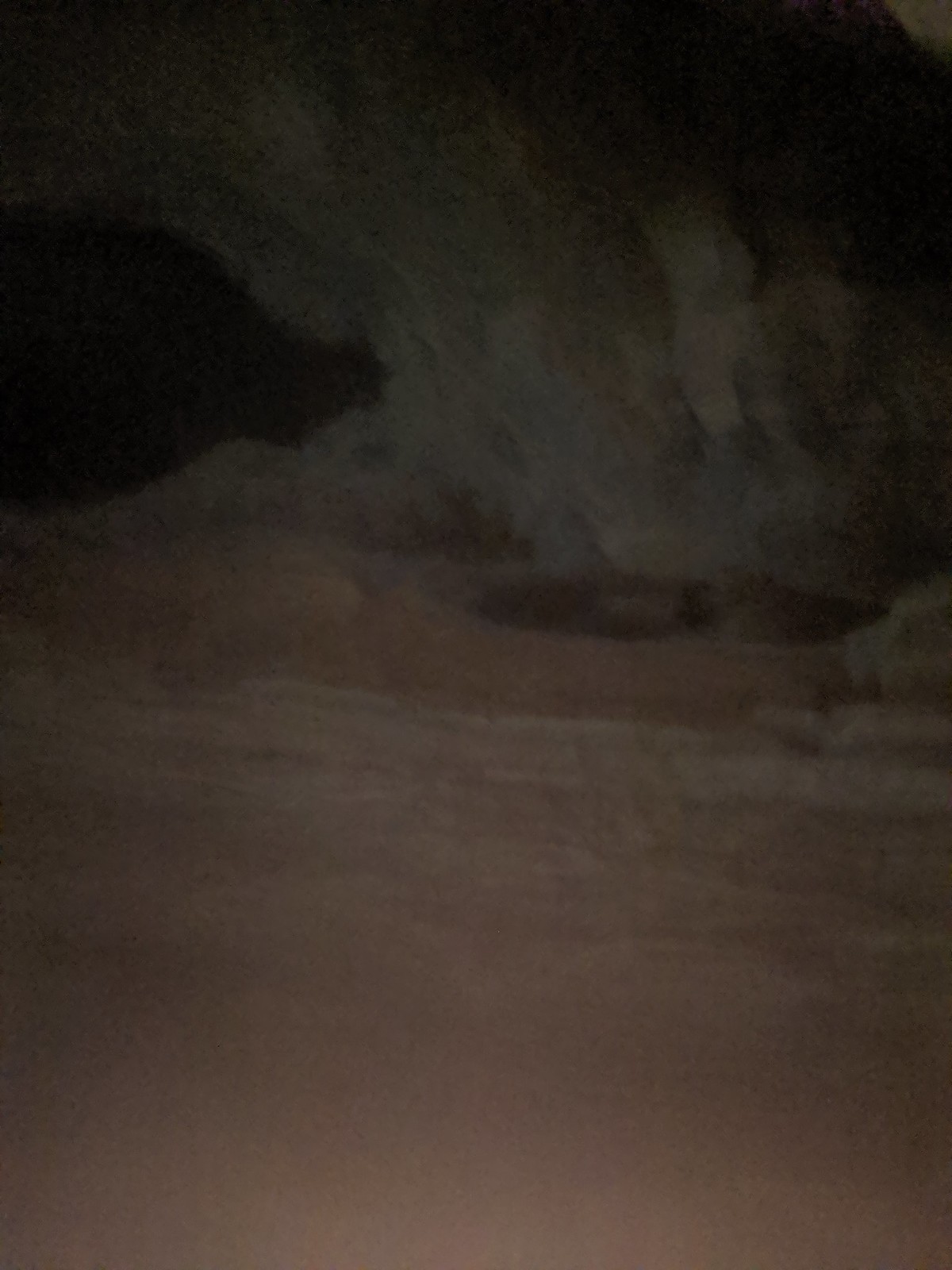The image depicts a cavernous scene with an intricate cave opening at its center. The base of the cavern floor is composed of a spectrum of tan hues, ranging from muted, light tans to deeper, darker tans. Dominating the scene is a crater-like hole that stands out with its darker shades concentrated on one side, adding depth and intrigue.

The focal point of the image is the cave entrance, which is shrouded in deep browns and blacks. This opening features a textured archway characterized by varying levels and rounded contours, creating a sense of depth and dimension. The colors within the image blend seamlessly together, producing a muted, unified palette that enhances the mystique of the scene.

Above the cave entrance, there is another darker shape, adding to the layered complexity of the cavern. The entire composition is devoid of any textual explanation, leaving viewers to interpret the enigmatic and atmospheric setting on their own.